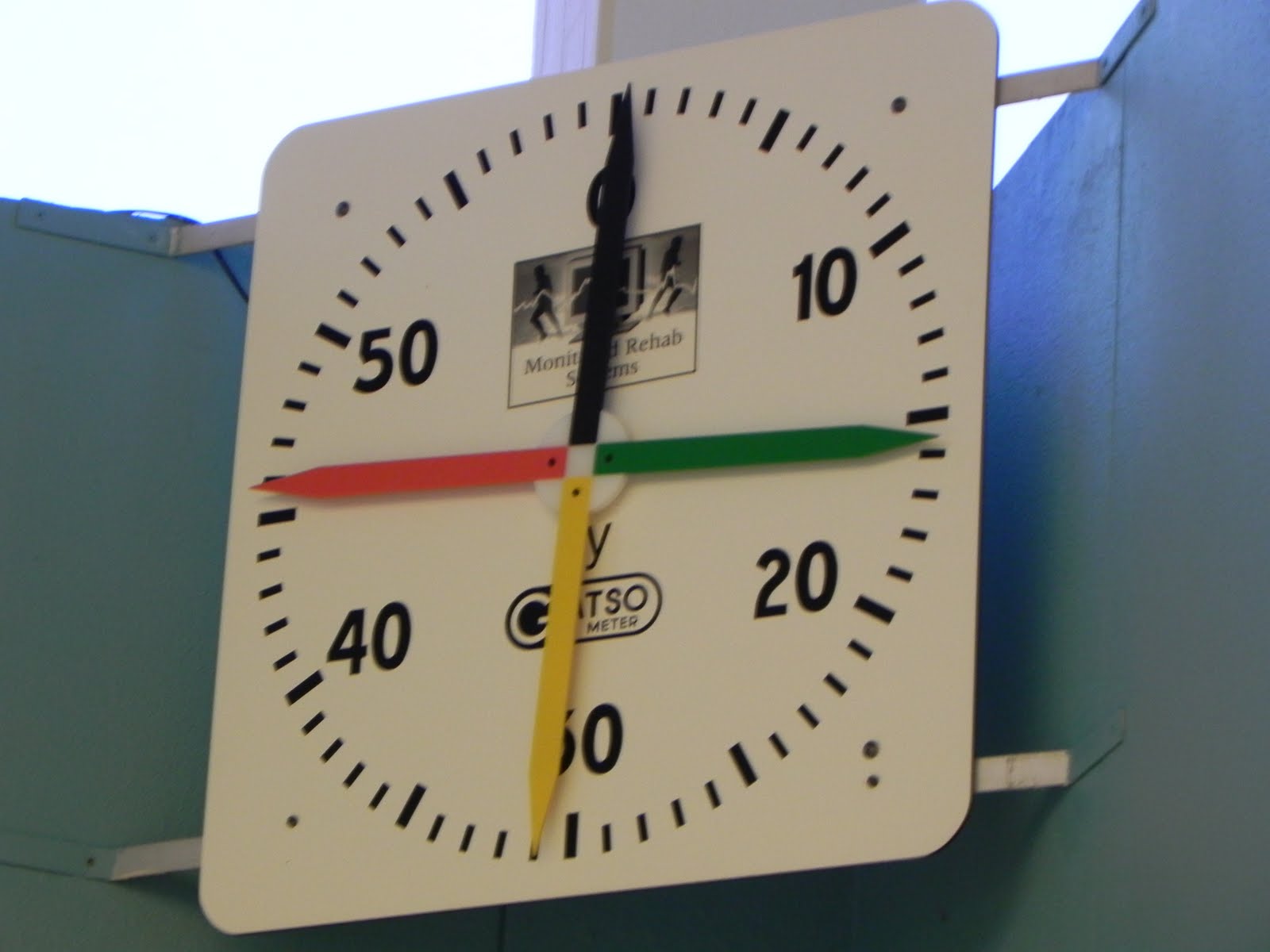This is a color photograph of an unusual, square-shaped device that resembles a clock, mounted in the corner where two light gray walls meet. The clock face is divided into increments from 0 to 50, and has four distinct hands: a black hand positioned at 0, a red hand around the 45 mark, a green hand near the 15 mark, and a yellow hand at approximately the 31 mark. A partially obscured logo appears near the top, depicting a computer terminal with lightning bolts emanating from it and two figures running away. The text accompanying this logo reads "Monitored Rehab Systems." Another logo is located near the 30 mark, but it is mostly hidden by the yellow hand. The visible part reads "system" and "meter."